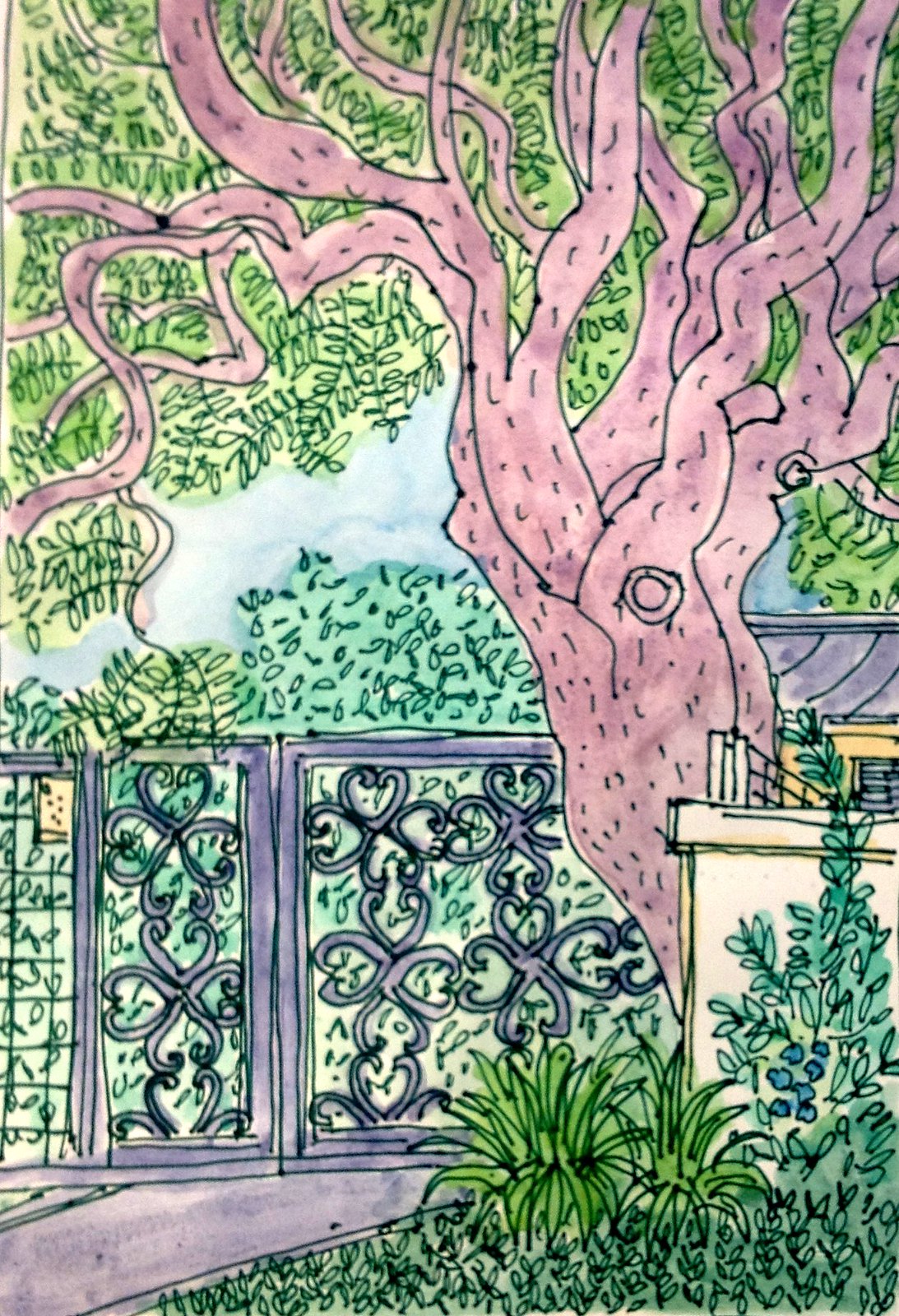This detailed illustration depicts the driveway of an affluent residence, characterized by a lush, green environment. Prominently, there's an old, richly textured tree with numerous ridges and bumps, its brown-reddish trunk and branches adorned with forest green leaves. To the right of the tree stands an ornate black metal gate with intricate bends and twists, leading into the driveway lined with various shrubs and bushes. In the background, partially obscured by the foliage, is a glimpse of a yellow house with a gray roof. The area is bordered by a tan, stucco-colored wall, enhancing the overall sense of affluence and seclusion. The artwork appears to be rendered using markers or watercolors, adding vibrant depth and detail to the scene.